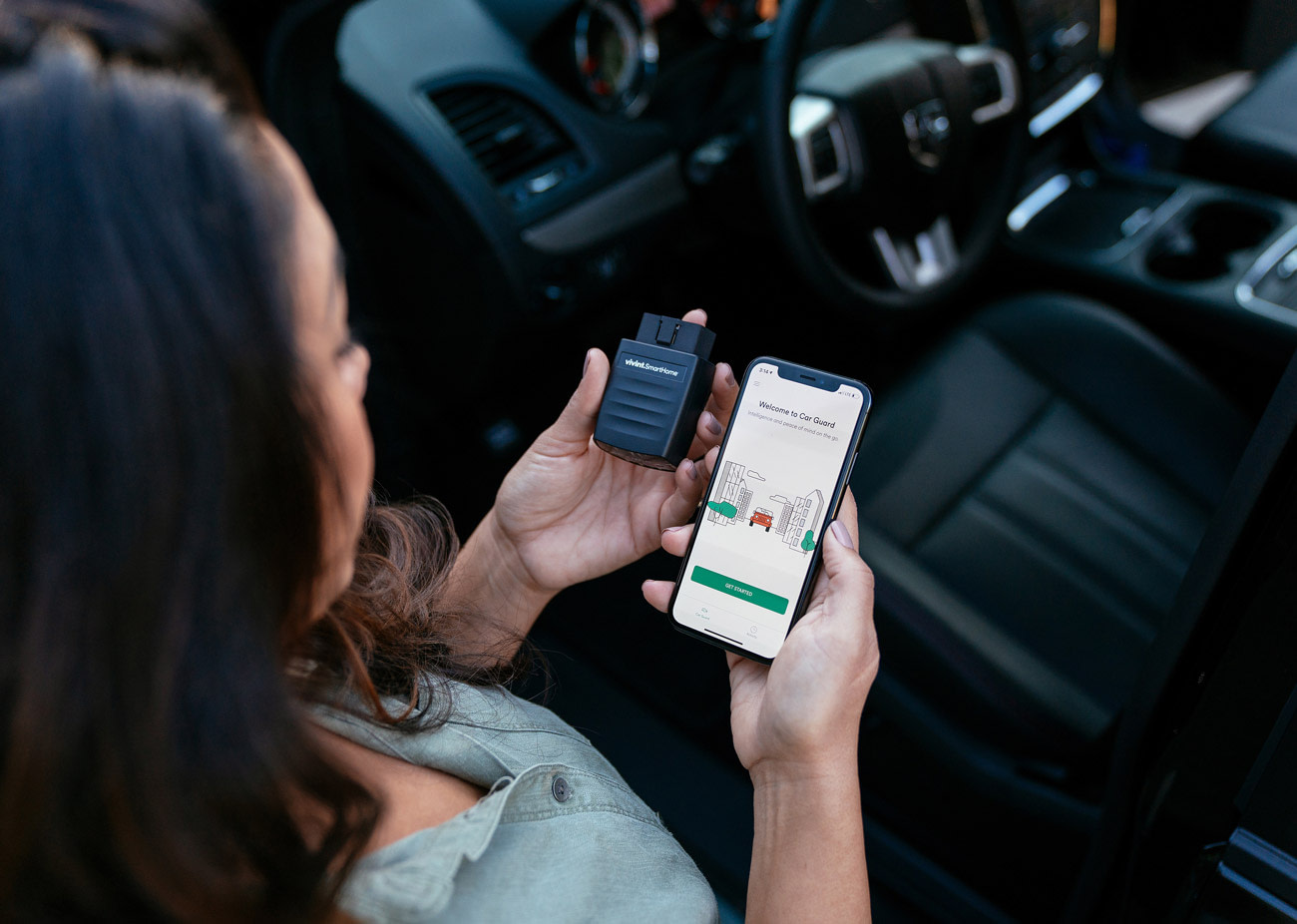The image depicts a woman with long, dark brown hair standing outside an open driver's side door of a car with a luxurious black leather interior, including detailed features such as cup holders, a black and silver steering wheel, and a center console. The woman, seen from behind, wears a light blue button-up shirt and holds a smartphone in her right hand displaying a message that says "Welcome to Car Guard." In her left hand, she grasps a black device, possibly a phone accessory or battery. The scene is detailed with vibrant colors including black, gray, green, red, and brown, and the setting suggests a staged photograph focusing on the intricate details of both the woman and the car.